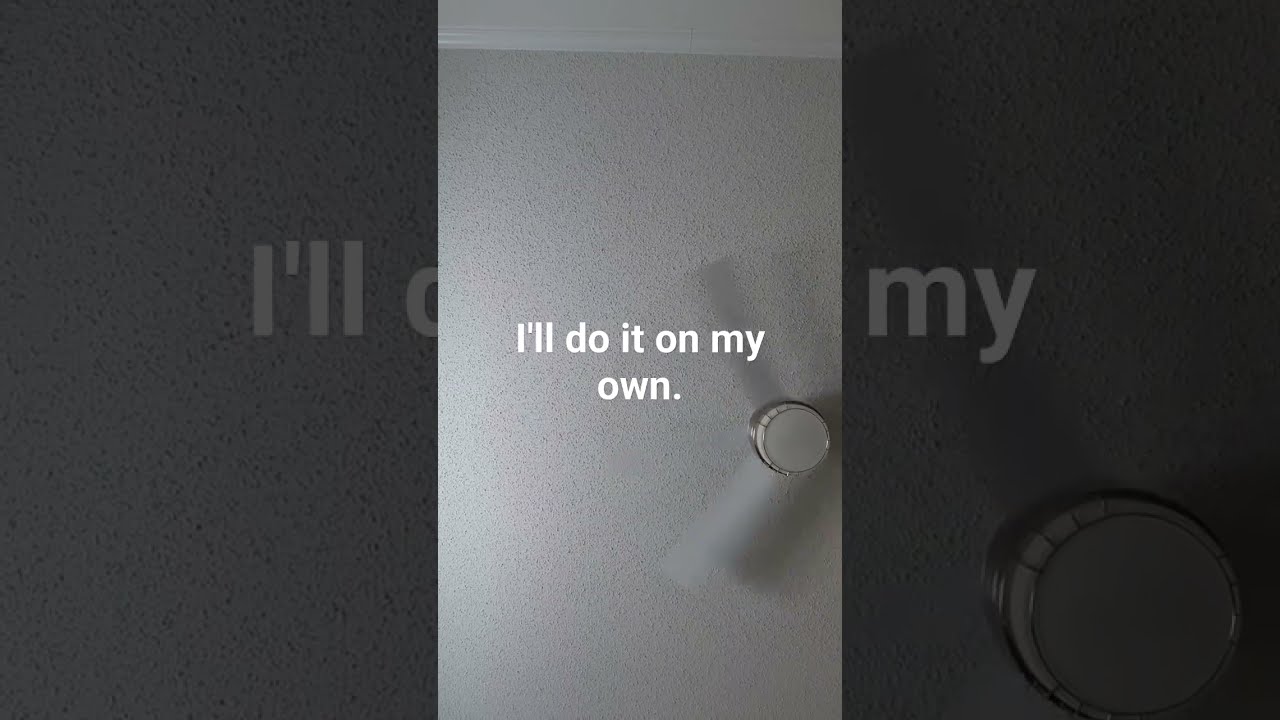In this striking image, a vertical cell phone photograph captures a textured, white popcorn ceiling. Positioned near the center, extending from the right edge, is a ceiling fan with two blurred blades, suggesting it is in motion. The fan features a flattened globe light encircled by a round silver trim and metal bars, though the light itself is not illuminated. Superimposed in the center of the image is a poignant message in white text, divided into two lines, reading "I'll do it on my own." This main photograph sits atop a horizontal background that is a zoomed-in, faded, and slightly blurry version of the same image, creating a layered effect with a dim, grayish tone.